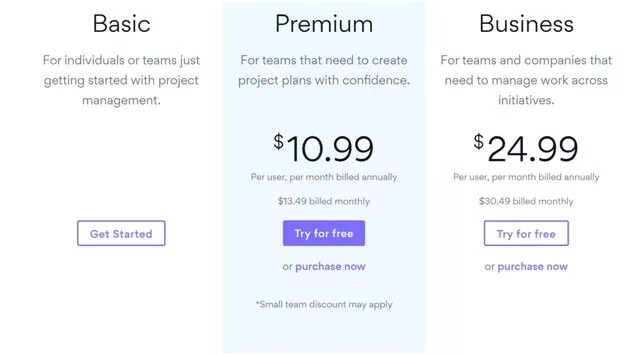In the image, there are three distinct categories for project management plans, each with a detailed description and a call-to-action button.

**Category 1: Basic**
- **Location:** Top left
- **Title Color:** Black
- **Description:** "For individuals or teams just getting started with project management."
- **Button:** A purple box with the text "Get Started."

**Category 2: Premium**
- **Location:** Top middle
- **Title:** "Premium"
- **Description:** "For teams that need to create project plans with confidence."
- **Price:** $10.99 per user per month (billed annually) or $13.49 per user per month (billed monthly)
- **Button:** A purple box with the text "Try for Free or Purchase Now."
- **Additional Info:** "Small team discount may apply."

**Category 3: Business**
- **Location:** Top right
- **Title:** "Business"
- **Description:** "For teams and companies that need to manage work across initiatives."
- **Price:** $24.99 per user per month

The image effectively categorizes different project management plans based on their functionalities and pricing, providing clear options for individuals, small teams, and larger companies.